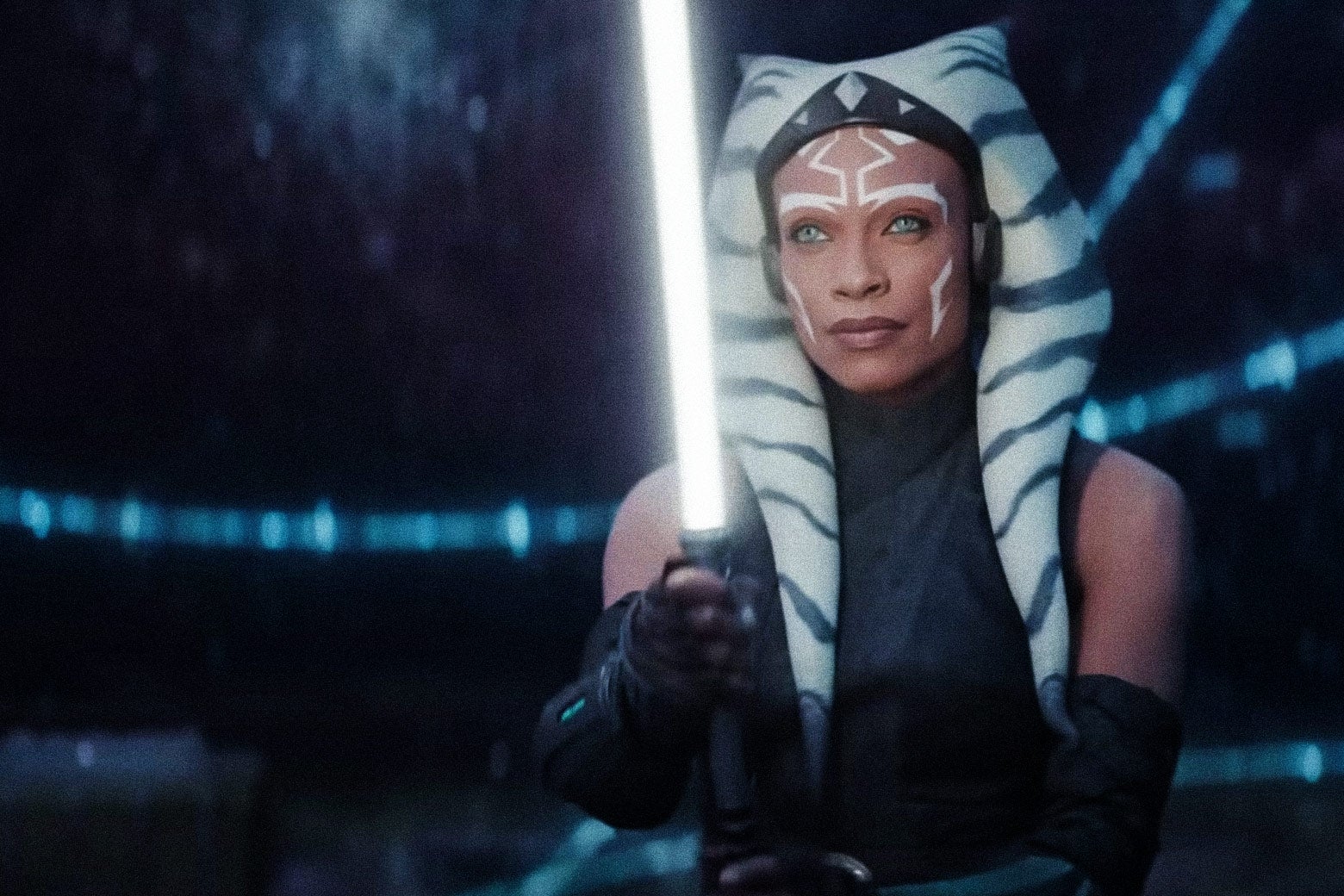The image features Ahsoka Tano, a prominent character from the Star Wars franchise, most notably appearing in the television show "Ahsoka." Positioned on the right-hand side of the photograph, Ahsoka is depicted from the waist up. She is instantly recognizable by her distinct facial markings, including white war paint with a partial diamond design on her forehead, and her striking blue eyes. Ahsoka wears a hat that resembles two striped legs extending down the sides of her head, akin to hair. She is dressed in a black, sleeveless top and long black gloves, with brown arms visible underneath. In her hands, she holds a lit white lightsaber.

The background is primarily dark, with black and deep blue hues, illuminated by a series of blue lights scattered throughout the scene, suggesting an otherworldly setting. The blue lights form a string running from the left-hand side, contributing to a slightly mysterious and futuristic ambiance. Ahsoka stands in a darkened room suffused with these blue accents, looking straight ahead with a determined expression.